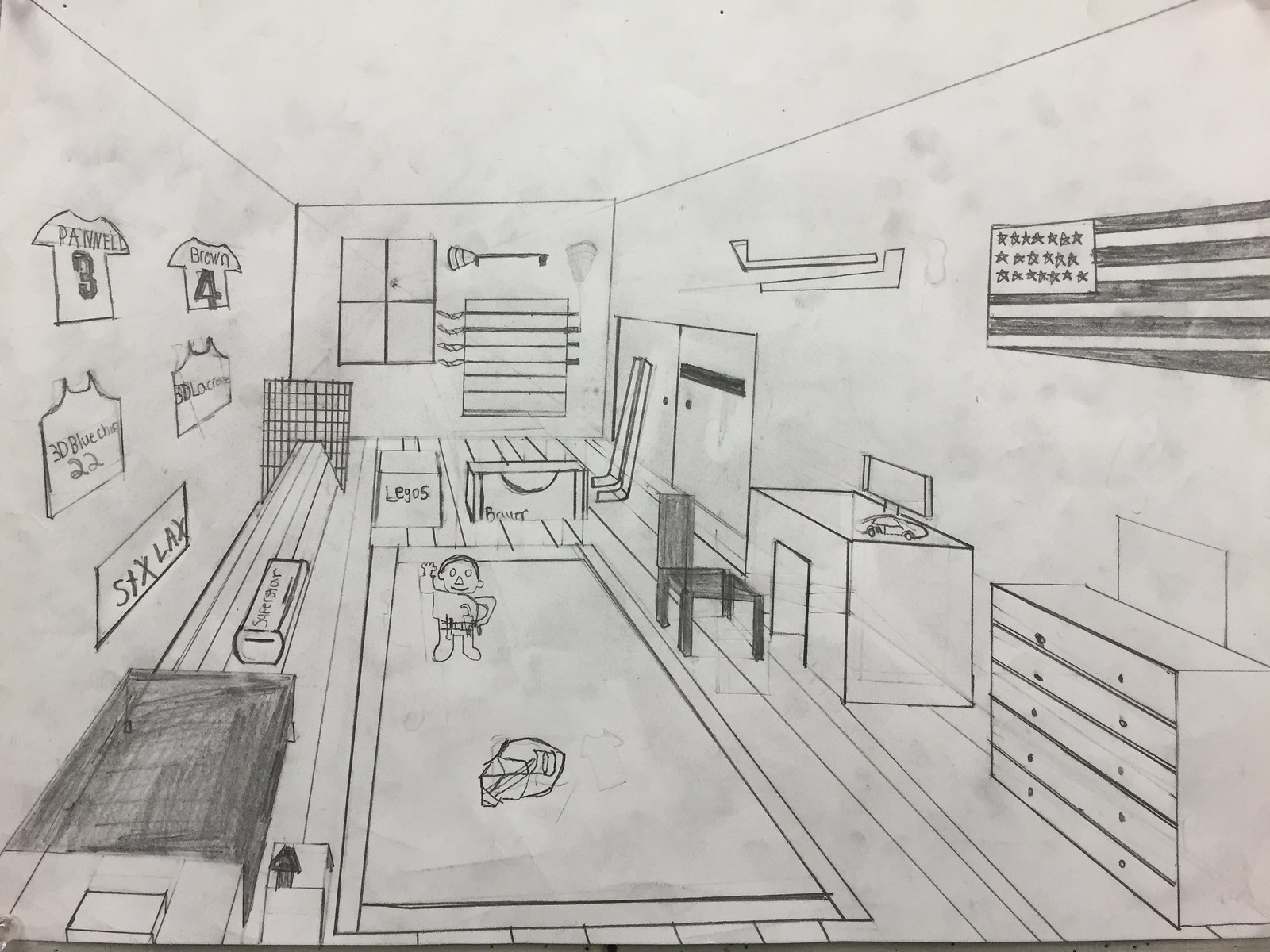This detailed illustration depicts a boy’s bedroom, carefully rendered in pencil, giving it a black-and-white appearance. The drawing adopts a perspective that converges toward the left-hand side, enhancing the depth within the room. In the middle, a small boy stands on an area rug, waving, and carrying a toy.

The room is filled with various items suggesting the boy’s interests. Surrounding him are boxes labeled "storage," scattered Legos, sneakers, and a helmet. The left wall features two jerseys, one labeled "Brown" and "Panthers 3" and the other "Blue Devils 22," signifying basketball and football themes. The right wall is adorned with an American flag, and notably, there are hockey sticks leaning against it.

A window graces the back wall, allowing a glimpse of natural light. The room is also furnished with a bed, a dresser, and a desk, which houses a computer and a toy car. Additionally, a lacrosse stick and related gear hint at another sport the boy might enjoy. The drawing, with its attention to dimension and detail, showcases the person’s skill in capturing the essence and personality of a lively and well-loved bedroom.